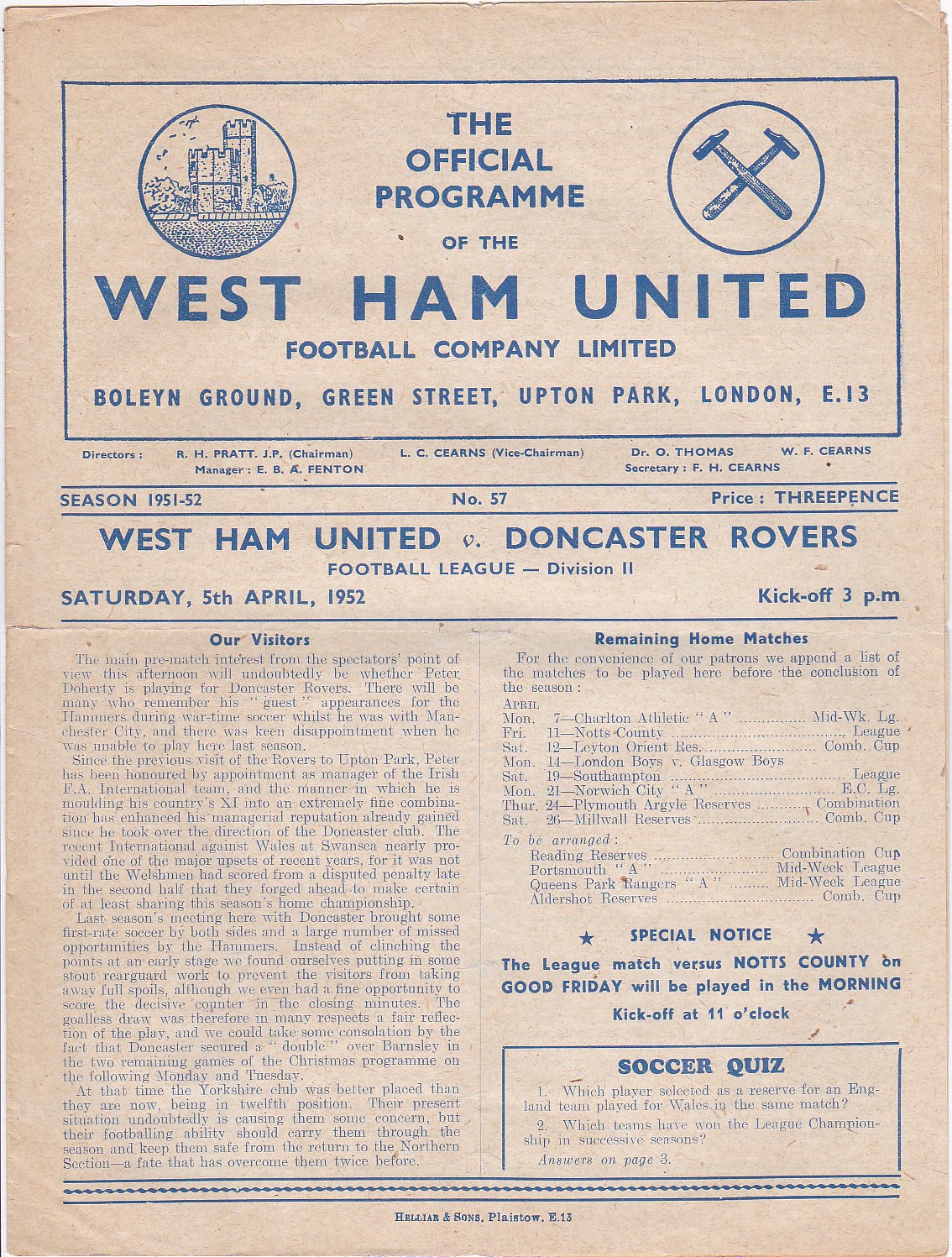The image depicts an old, worn-out flyer, likely from the 1951-52 season, related to soccer leagues, specifically West Ham United. The background, once white, now appears brown due to age. At the top of the flyer is a blue-bordered box containing the title "The Official Program of the West Ham United Football Company Limited," with the address "Boleyn Ground, Green Street, Upton Park, London, E.13" at the bottom of the box. On the left side of this box is a blue circle with a castle drawing, while the right side has a blue circle featuring two crossed hammers.

Below this top section, the flyer lists the season "1951-52" and identifies the issue as "Number 57" with a price of "3 Pence." The main content announces the match: "West Ham United vs. Doncaster Rovers, Football League, Division II," with a kickoff time of "3 p.m." on "Saturday, 5th April 1952." On the left side, a section titled "Our Visitors" likely details the visiting team, though the text is too worn to read clearly. The right side lists "Remaining Home Matches" with various dates and opponents. Toward the bottom, there is a "Special Notice" about the League Match against Knotts County being played on Good Friday morning at 11 o’clock. In the bottom right corner, there's a section titled "Soccer Quiz."